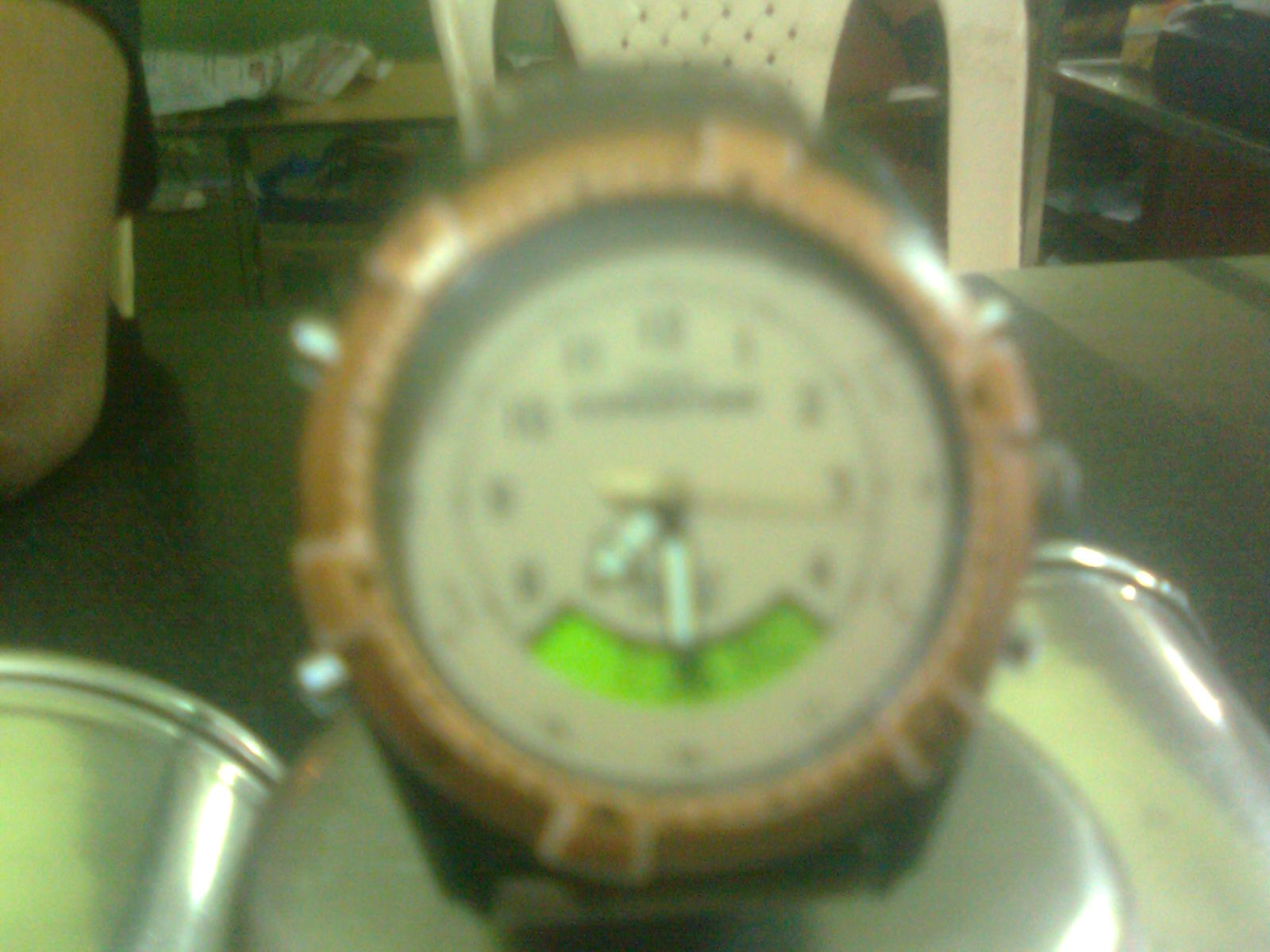This color photograph, taken indoors under artificial light, features a prominently centered analog watch, exuding a distinct yellowish-green tone, possibly due to a filter. The image appears blurry and grainy, with noticeable light beams hitting the subject. Dominating the scene, the watch has a medium brown plastic or wooden bezel and a cream-colored face. Black numbers encircle the face, though they are hard to read due to the blur. Notably, a green LCD screen occupies the lower section between numbers 5, 6, and 7. Silver watch hands, with a gold second hand pointing just past 3, indicate the time is 7:30. The watch rests on a possibly metal or stainless steel surface, possibly a scale, accompanied by another metallic object to its left. In the background, a white perforated plastic chair and a brown upholstered piece of furniture are visible, alongside a gray tabletop on which the watch and objects are placed. Additionally, the upper left corner hints at a partial figure, while the upper right reveals steps, pointing to a cluttered indoor setting.